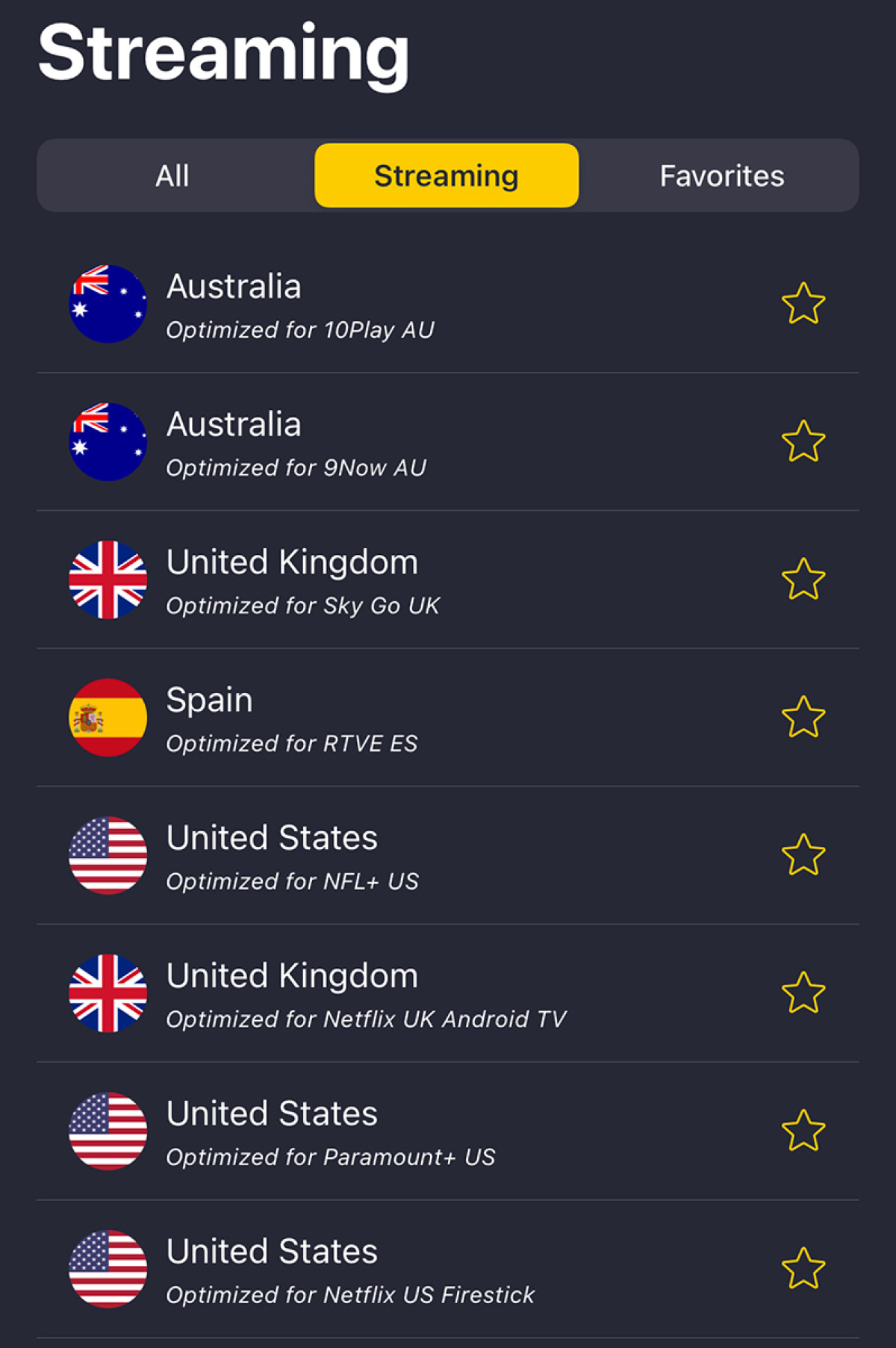Caption: The image showcases a user interface of a streaming service with three tabs labeled "All," "Streaming," and "Favorites." The "Streaming" tab is highlighted in yellow, indicating it is currently selected. Below the tabs, a list of streaming options is displayed, each prefaced by a small star icon that is not filled in, suggesting they have not been marked as favorites. The options are:

1. Australia - Optimized for 10 Play AU
2. Australia - Optimized for 9Now AU
3. United Kingdom - Optimized for Sky Go UK
4. Spain - Optimized for RTVE (ES)
5. United States - Optimized for NFL+ US
6. United Kingdom - Optimized for Netflix UK Android TV
7. United States - Optimized for Paramount+ US
8. United States - Optimized for Netflix US Fire Stick